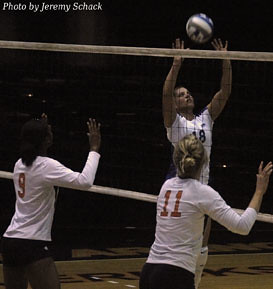In this detailed photograph of a women's volleyball game, three female players are captured mid-action. The focal player, wearing the number 18 on her white jersey with black lettering, is in mid-air, her hands poised to set the white and blue volleyball. Her hair is pulled back, emphasizing her focus and athleticism. Opposite her, across the net, are two defenders readying themselves to jump and block the impending set. The defender on the left, an African-American player, sports the number 9 on her white jersey with red numbers, while the Caucasian player on the right wears the number 11. Both defenders also have their hair pulled back and are attired in white jerseys with black shorts. In the top left corner of the image, the credit reads "Photo by Jeremy Shack."